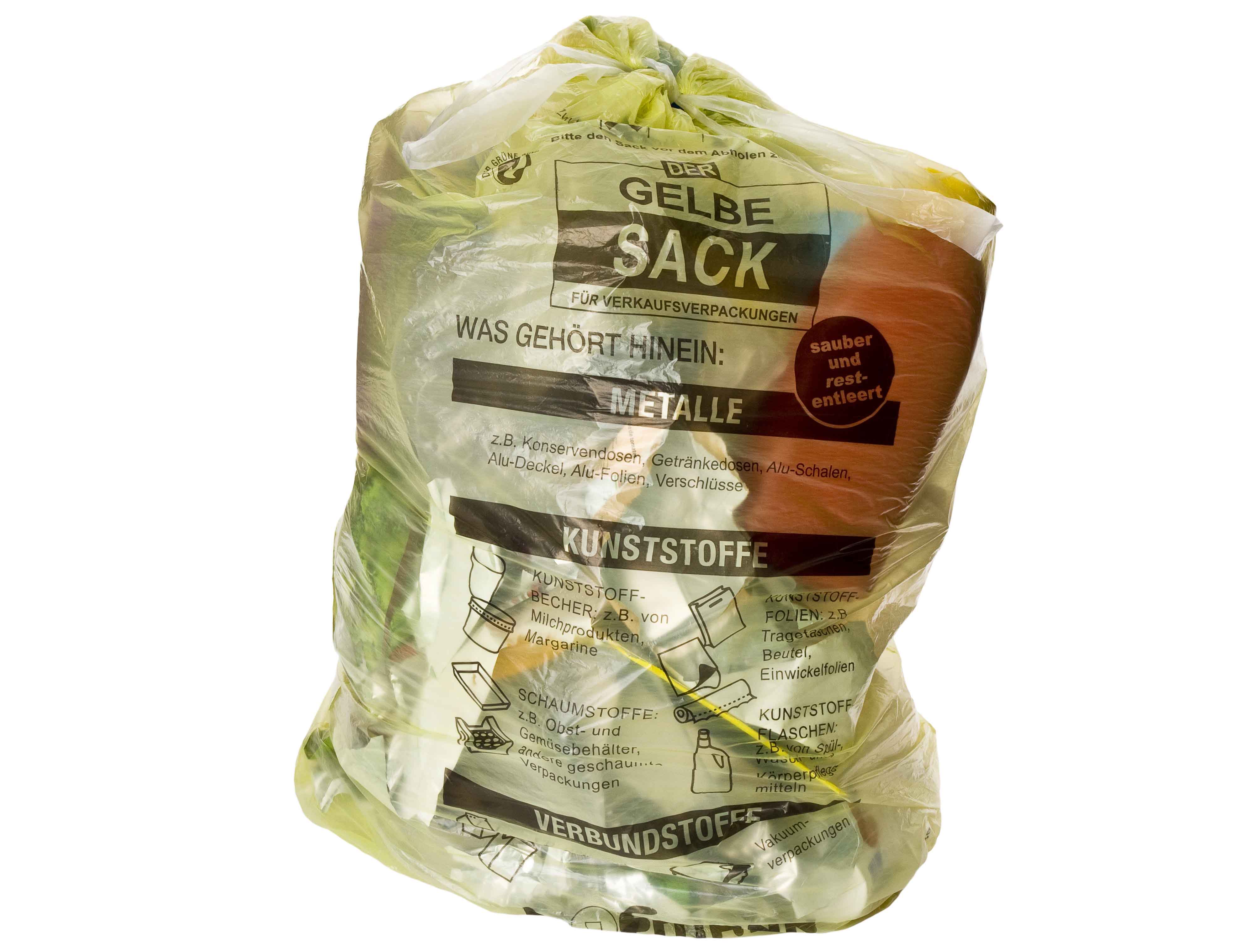The image depicts a partially transparent plastic bag with a yellowish tint, filled to capacity with various waste items. The bag is tied at the top and features extensive German text in black. The top of the bag prominently displays the title "Gelbe Sack" in a black rectangle, followed by the long phrase "Für Verkaufsverpackungen." Below this, there are three sections labeled "Metall," "Kunststoffe," and other categories, each with symbolic depictions, such as a detergent bottle, trash cans, baking pans, and plastic bottles. Additionally, some visible items inside the bag include a white envelope and a reddish-orange bottle. The text serves as a guideline on what materials can be placed in this recycling bag.